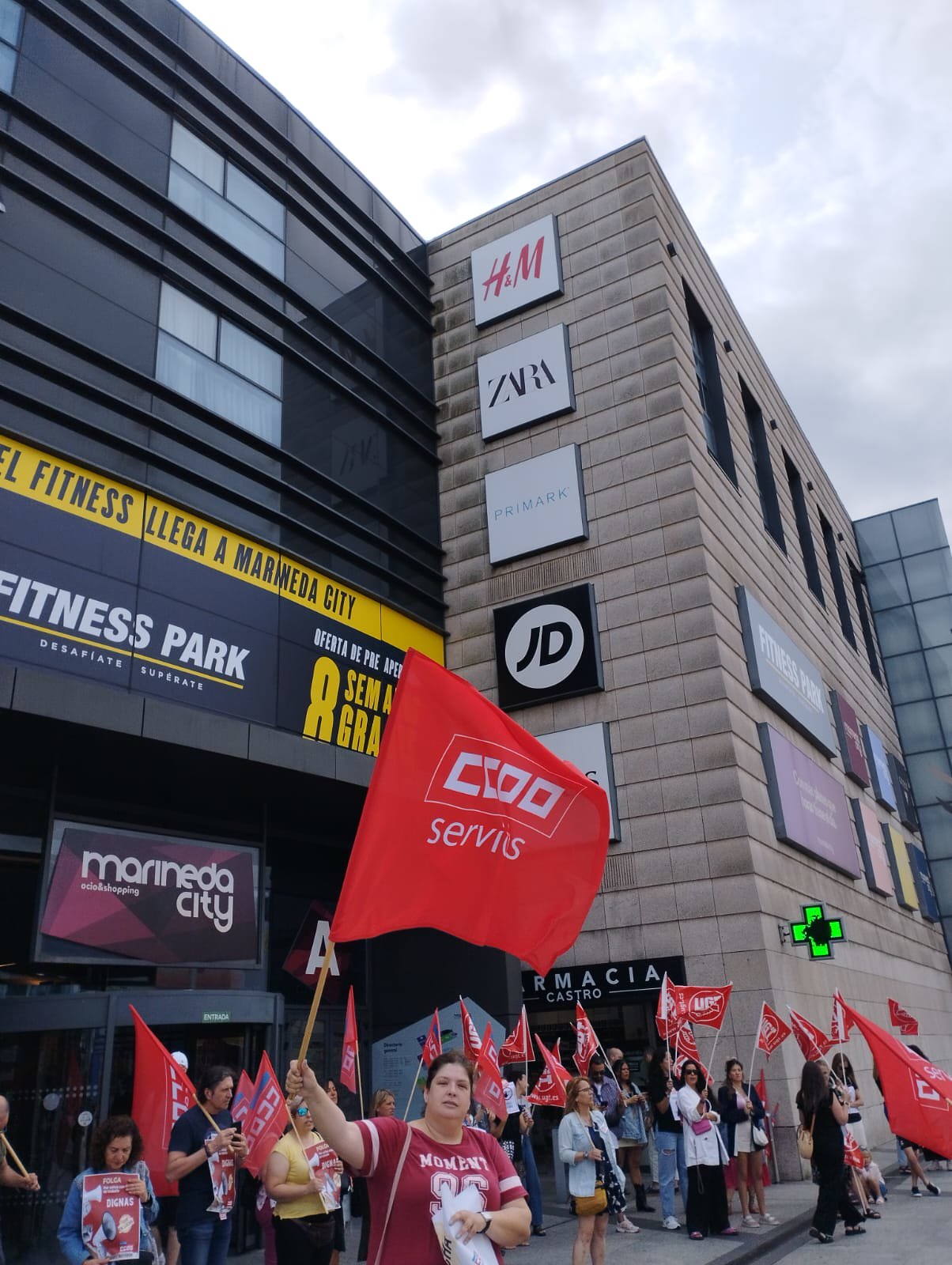In a vibrant outdoor scene on a sunny day with a few scattered green-gray clouds, a bustling street in front of a three-story building is the setting for a vivid display of activism. The photograph captures a group of predominantly women engaged in what appears to be a protest. They are holding red or orange flags bearing the white text “COOSERVIS.” At the forefront, a prominent woman in a red t-shirt with white markings is energetically waving her flag. Alongside her, around 20 other women are gathered on the sidewalk, waving flags and holding signs, each dressed distinctively -- from a woman in a white jacket and black pants, to another wearing a black jacket and a white skirt, and another sporting a blue jacket over a black dress. A woman in a yellow tank top and black pants stands out, as does another in a blue jacket, who is holding a sign.

The backdrop features an assortment of signs and logos on the building behind them, indicating a commercial area or a shopping mall. The signs read "Maranata City Fitness Park," "Fitness LLEGA," "A Maranata City," "ASMAGRA," "JD," "ZARA," "H&M," and "Primark," among others, suggesting a significant shopping district, likely in a Spanish-speaking country. The scene is bustling with activity, with the women's unity and spirited presence dominating the photograph.